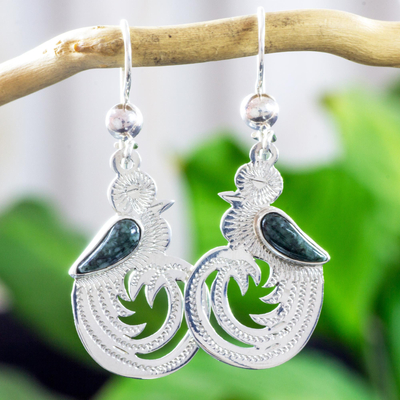The image depicts a pair of large, detailed earrings, intricately designed to resemble birds. Each earring is made primarily of sterling silver or a similar light-colored metal, meticulously sculpted to represent a bird facing its counterpart. Their bodies and heads are elegantly shaped, featuring a circular ball atop each head and an elaborate, swirly tail that completes the bird's form in a full circle.

Attached separately to their bodies, the wings are crafted from a dark, blackish-blue stone, providing a striking contrast to the rest of the silver structure. Both earrings are mirror images of each other and are suspended from silver hooks. They hang delicately from a thin pine branch, set against a blurry green background that suggests an outdoor setting. The overall appearance is both refined and natural, capturing the essence of avian beauty and elegance.